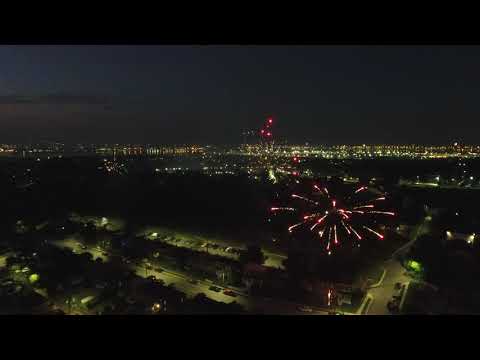This nighttime photograph captures a dazzling firework display set against an urban backdrop. The foreground features a roadway illuminated by streetlights, with a few cars parked along its sides. The cityscape beyond is brightly lit, indicating a large metropolitan area. The sky is dark, with a slightly hazy patch to the left. Two prominent red fireworks dominate the scene, one nearer and another farther in the distance, while additional fireworks are visible as red dots, either pre-explosion or as part of the ongoing display. The ground beneath the fireworks showcases silhouetted trees, and whether there's a body of water remains ambiguous due to the darkness. The overall scene suggests a festive celebration, highlighted by the vivid contrasts of vibrant fireworks against the serene night sky and the shimmering city lights.